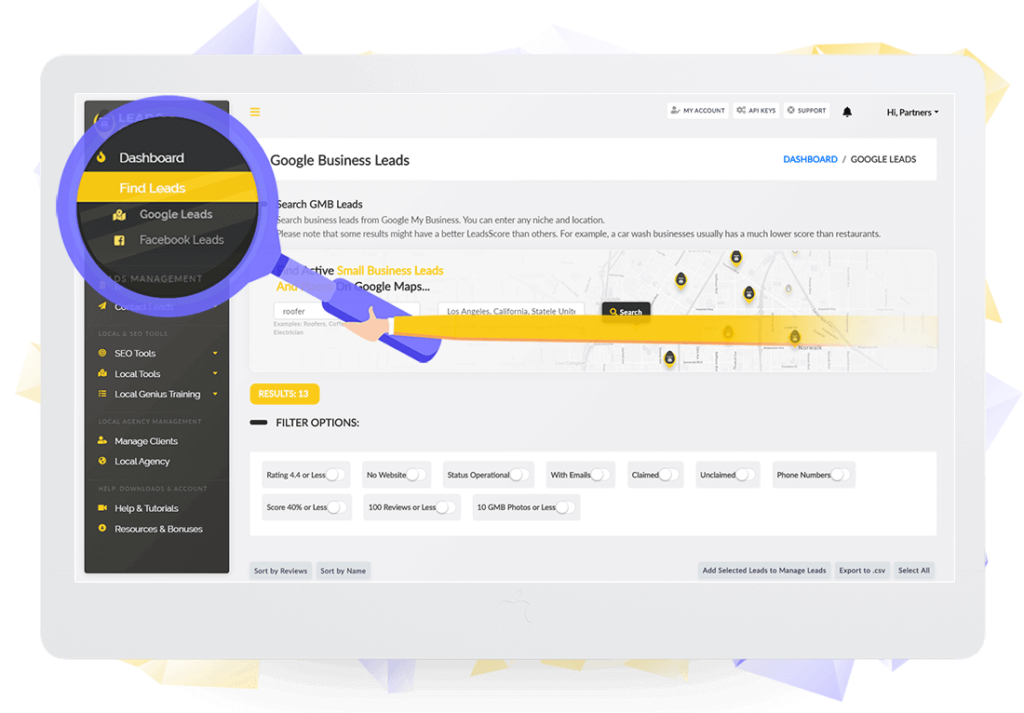The image is a screenshot of a computer screen displaying a dashboard interface of a lead management tool. The overall background is gray, with a prominent central box containing various elements. On the left side of this box, there is a vertical black rectangular panel listing several menu items such as "Dashboard," "Find Leads," "Google Leads," "Facebook Leads," and an item labeled as "Something Management." 

Below these items, "Dashboard" is highlighted by a blue magnifying glass icon, with an illustrated hand extending toward it. Beneath this section, the menu continues with additional options like "SEO Tools," "Local Tools," "Local Genius Training," "Manage Clients," and "Local Agency."

The central portion of the screen is filled with text and features a map. The text prominently displays "Google Business Leads" and "Dashboard Google Leads." The map has several black markings, presumably indicating the locations of businesses of interest. Additionally, there are options to filter the displayed leads, enhancing the usability of the tool.